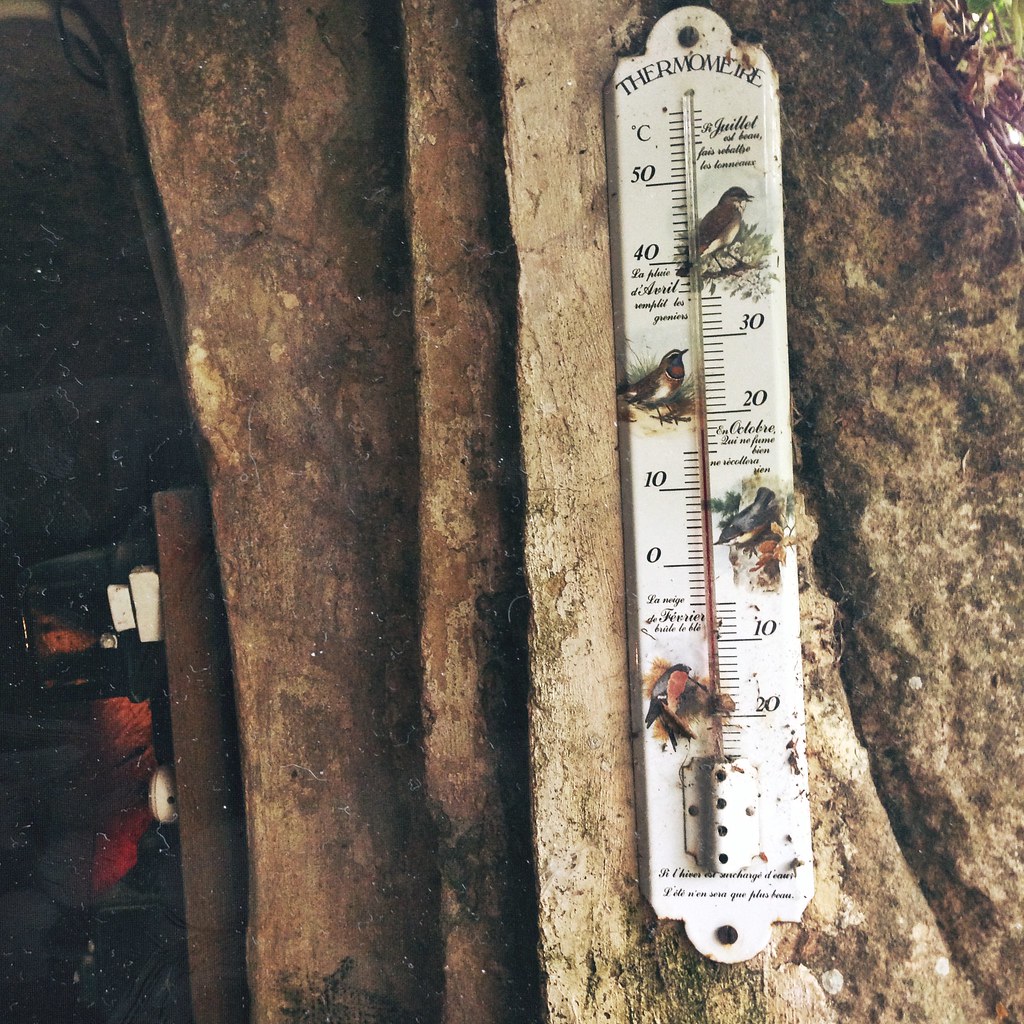This artwork appears to be a painting depicting a close-up view of a large tree trunk, to which a vintage thermometer is affixed. The thermometer, reminiscent of a white ruler, is prominently displayed, with detailed markings indicating temperatures ranging from 20 to 50 degrees Celsius. This instrument features a classic glass tube filled with red liquid to measure temperature changes. Adorning the edge of the thermometer are illustrations of four different birds, each presumably labeled with descriptions too small to discern. The background to the left of the tree fades into an indistinct dark area, interspersed with hints of red and two small rectangular white shapes. The overall texture and appearance of the painting suggest an antiquated look, achieved through subtle speckling and splattering of white paint, mimicking the aesthetic of an old photograph.